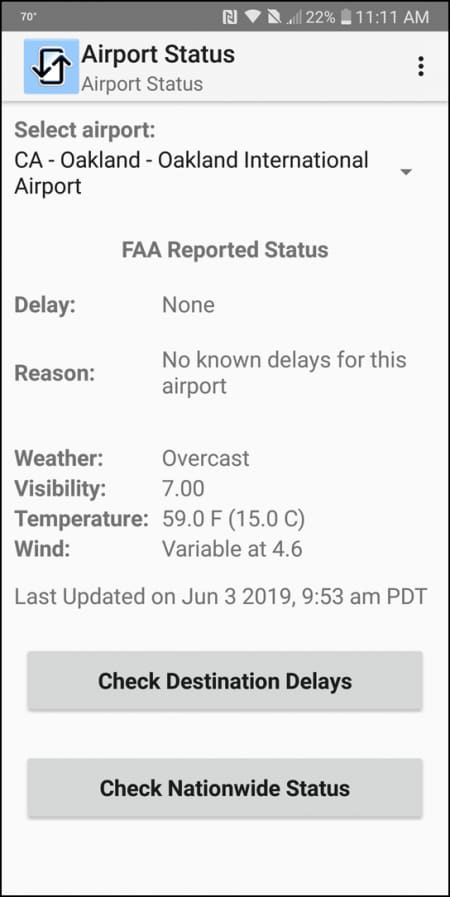**Detailed Caption:**

This is a detailed screenshot captured from a mobile phone. At the very top of the screen, there is a gray status bar containing various pieces of information displayed in white text. On the far left of the bar, it shows the temperature as 78 degrees. Moving towards the right, there are several icons: a full Wi-Fi signal indicator, an SD card symbol, a mobile signal meter indicating one out of five bars, and a battery icon showing a 22% charge level. The time is displayed as 11:11 a.m.

Below the status bar, the main content starts on a white page. At the top of this page, there's a small icon featuring two arrows forming a rectangle against a blue background, indicating some form of status display. Next to this icon, in black font, it reads "Airport Status," followed by the same text in gray font below it as a subtitle. Positioned to the right of this text are three vertically aligned black dots, suggesting a menu or additional options.

A gray bar divides this header from the main content below. Underneath, the text reads "Select Airport, CA-Oakland-Oakland International Airport," followed by "FAA Reported Status." The detailed report states: 
- Delay: None
- Reason: No known delays for this airport
- Weather: Overcast
- Visibility: Seven miles
- Temperature: 59 degrees Fahrenheit (15 degrees Celsius)
- Wind: Variable at 4.6 mph

The information concludes with a timestamp, indicating that the data was last updated on June 3, 2019, at 9:53 a.m. PDT.